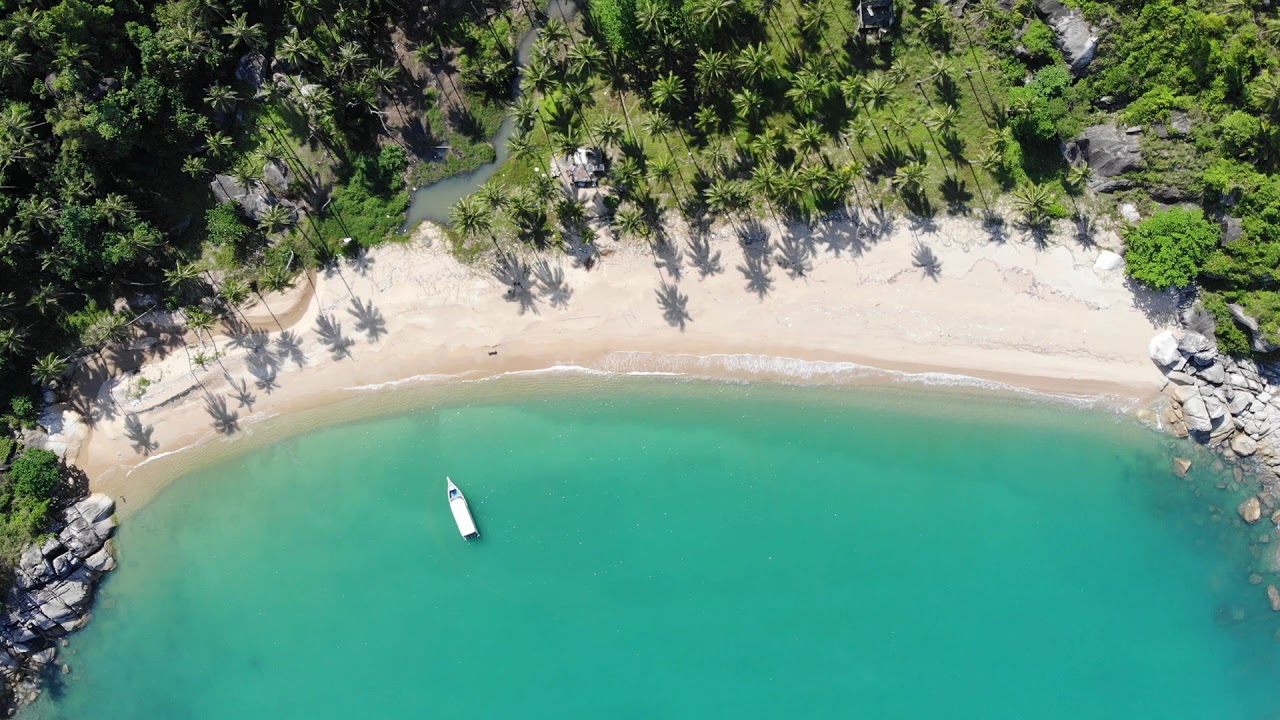This horizontal rectangular photograph, taken from a drone or helicopter, captures a stunning aerial view of a pristine beach. The foreground reveals clear, turquoise waters that seamlessly transition into sandy shores. You'll notice an intriguing white object floating in the bottom left of the water, resembling a small boat.

The middle of the image features an expansive sandy beach area punctuated by numerous scattered boulders and a variety of lush greenery, including an abundance of trees and palm trees. On the far left, there are some larger rocks, while scattered white boulders frame both the left and right edges where they meet the water. Along the left side, you can also see several chairs positioned for a perfect view of the serene waters. 

In the background, a dense tapestry of mixed trees, including numerous palms, creates a vibrant, green backdrop. The entire setting epitomizes a tranquil, typical beach environment, blending the natural beauty of sand, water, and foliage.